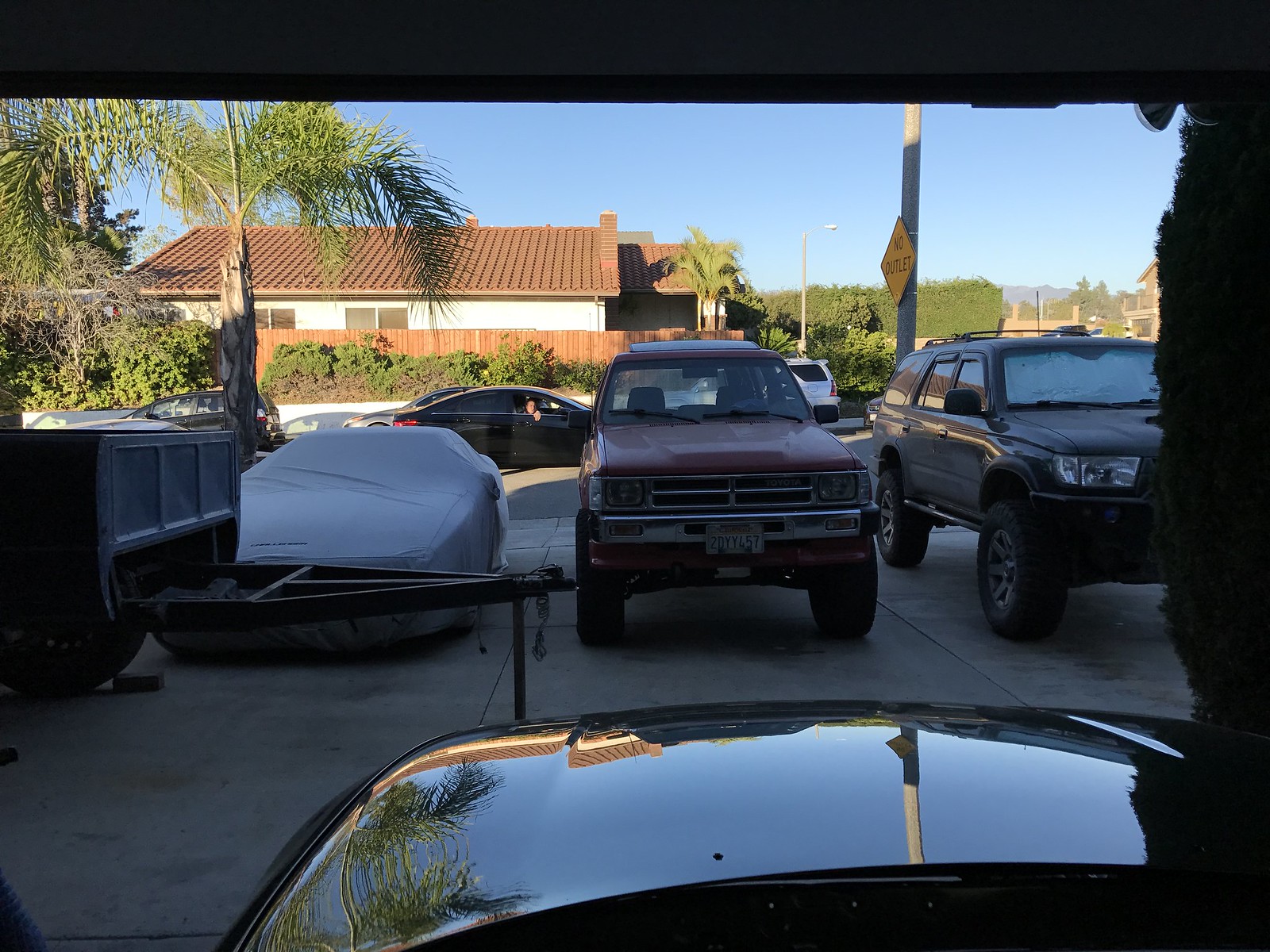A bright outdoor photograph captures a large driveway and the street beyond it. The image is taken from inside a garage, looking over the glossy, reflective hood of a dark car, which mirrors an adjacent tree. At the end of the driveway, a house with a clay-colored roof is visible under a clear blue sky. Various vehicles populate the scene: directly in front, there's the black end of a pickup truck with a hitch. To the right, a newer dark SUV is parked near a tall, dark bush. A red, older-style Mazda truck is positioned to the left, near a small sports car that is partially covered with a white car cover. Further to the left, there's a blue dumpster. On the road, a black car drives by with a person looking toward the photographer. A "no outlet" sign on a yellow triangle sits atop a utility pole behind the SUV. The overall scene is vibrant with details like the palm tree to the left and the asphalt driveway lined with various parked and passing cars.